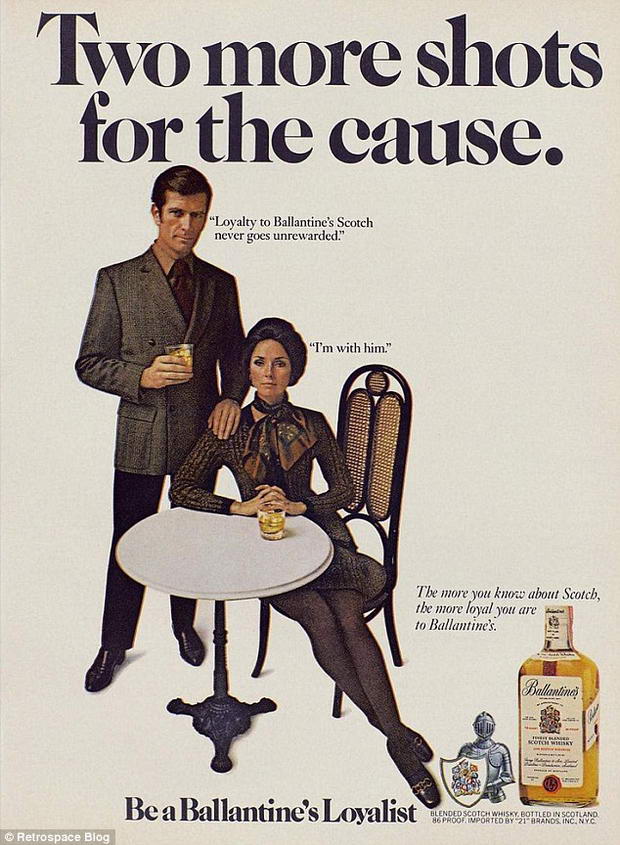The image is a vertical rectangular advertisement, likely from an old magazine, promoting Valentine's Scotch whiskey. Central to the image are a distinguished man in a brown suit, standing behind a woman who sits somewhat sideways on an ornate chair at a small round table. Both hold glasses of Scotch, hers resting on the table, while his is in his right hand with his left hand gently placed on her shoulder. The background is beige, giving the scene a vintage feel. 

At the top of the advertisement, bold black letters proclaim, "Two more shots for the cause." Just below, more text emerges, with phrases such as "loyalty to Valentine's Scotch never goes unrewarded" and "I'm with him." The bottle of Valentine's Scotch whiskey, accompanied by additional promotional text such as "Be a Valentine's loyalist" and details about the Scotch's origins and importer, is positioned in the lower right corner. Near this bottle, an illustration of a knight in armor standing with a shield accentuates the advertisement's regal and timeless appeal. The overall palette features tones of white, black, gold, gray, and brown, enhancing its classic ambiance.